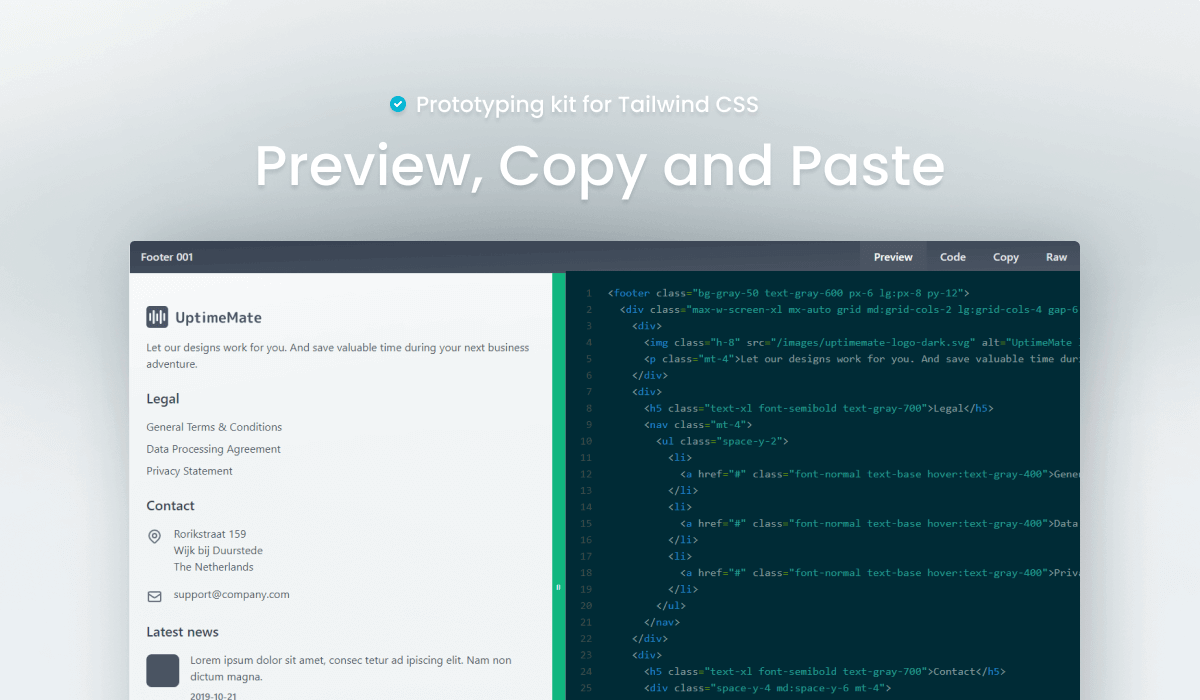The image is a screenshot from a web page with a whitish green, cloudy background. At the top of the image, there's text that reads "A prototyping kit for Tailwind CSS" and below it, in larger white font, "Preview, copy, and paste". The bottom section of the image features a rectangular footer divided into black on the right side and white on the left side. 

On the white left side:
- The text "Footer 001"
- The section "Uptime Mate" with the tagline "Let our designs work for you and save valuable time during your next business adventure."

Under the "Legal" section:
- "General terms and conditions"
- "Data processing agreement"
- "Privacy statement"

In the contact section:
- An icon of a pin followed by the address: "Rorastat 159 Wijkje Bija Durenstede, the Netherlands"
- An envelope icon indicating an email option with the address "support@company.com"

Additionally, there is a "Latest News" section, though the text in this part appears to be in a difficult-to-read foreign language.